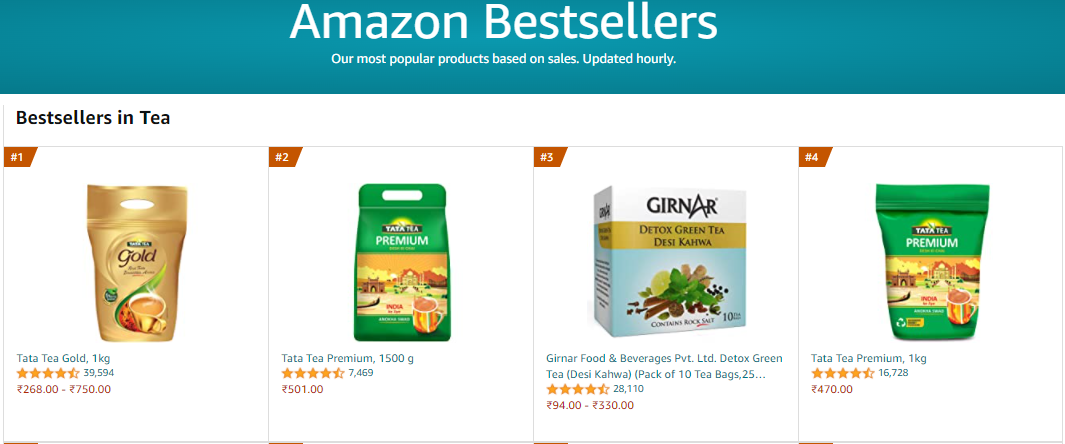The top section of the page features a teal background with prominent white text that reads, "Amazon Bestsellers." Below this heading, in smaller white text, it states, "Our most popular products based on sales. Updated hourly." 

On the left side, in black text, it announces, "Bestsellers in Tea." Ranked number one is a gold package displaying a cup of red-colored liquid, with a green leaf positioned behind it. Beneath the image, the text reads, "Tata Tea Gold, 1 kilogram," with a price range of ₹268-750.

Ranked at number two is "Tata Tea Premium," presented in a green container with a depiction of a tea mug on its front. The listed price for this item is ₹501.00.

To the right of this, there is a product in a blue container featuring images of spices and leaves on its front. This product is labeled "Detox Green Tea," and its price ranges from ₹94 to ₹330.

Lastly, within the rankings, there is another "Tata Tea Premium" in the identical green container as the second item. However, the price for this entry is marked at ₹470 in red text.